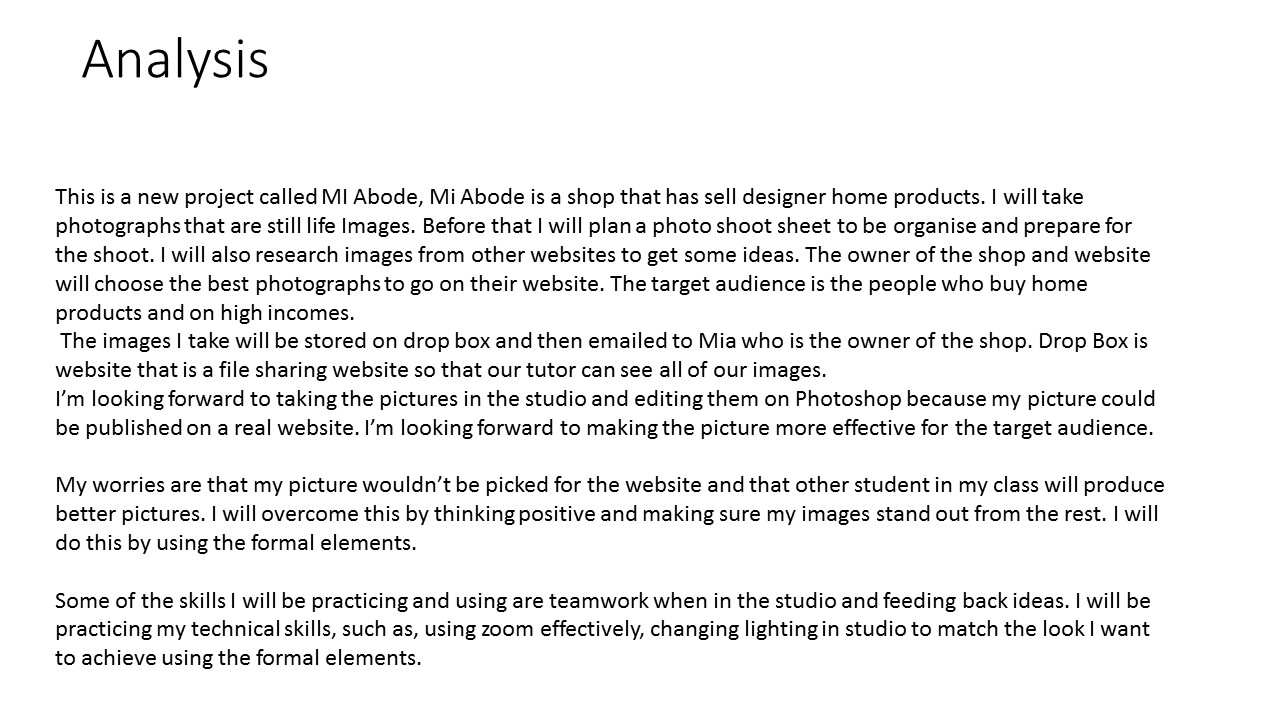The image appears to be a screenshot or photo of a PowerPoint slide from a presentation. The slide features a white background with only black text, and no images, color, or clip art. The title of the slide, located in the top left corner, reads "Analysis." Below, the slide discusses a new project called "MI Adobe," which involves a shop that sells designer home products. The text details the plan for photographing still-life images of the products, including steps for organizing a photoshoot, researching ideas from other websites, and having the shop owner choose the best photos for the website. The target audience is affluent individuals who purchase home products. The images will be stored on Dropbox and emailed to Mia, the shop owner. The presenter expresses excitement about taking and editing photos in the studio, aiming to make the pictures effective for the target audience. The slide also mentions concerns about other students producing better images and overcoming those worries by thinking positively and ensuring the photos stand out. Key skills to be practiced include teamwork, technical aspects of photography like zoom and lighting, and the application of formal elements. The presenter seems to have prepared thorough notes that might guide them during their spoken presentation.